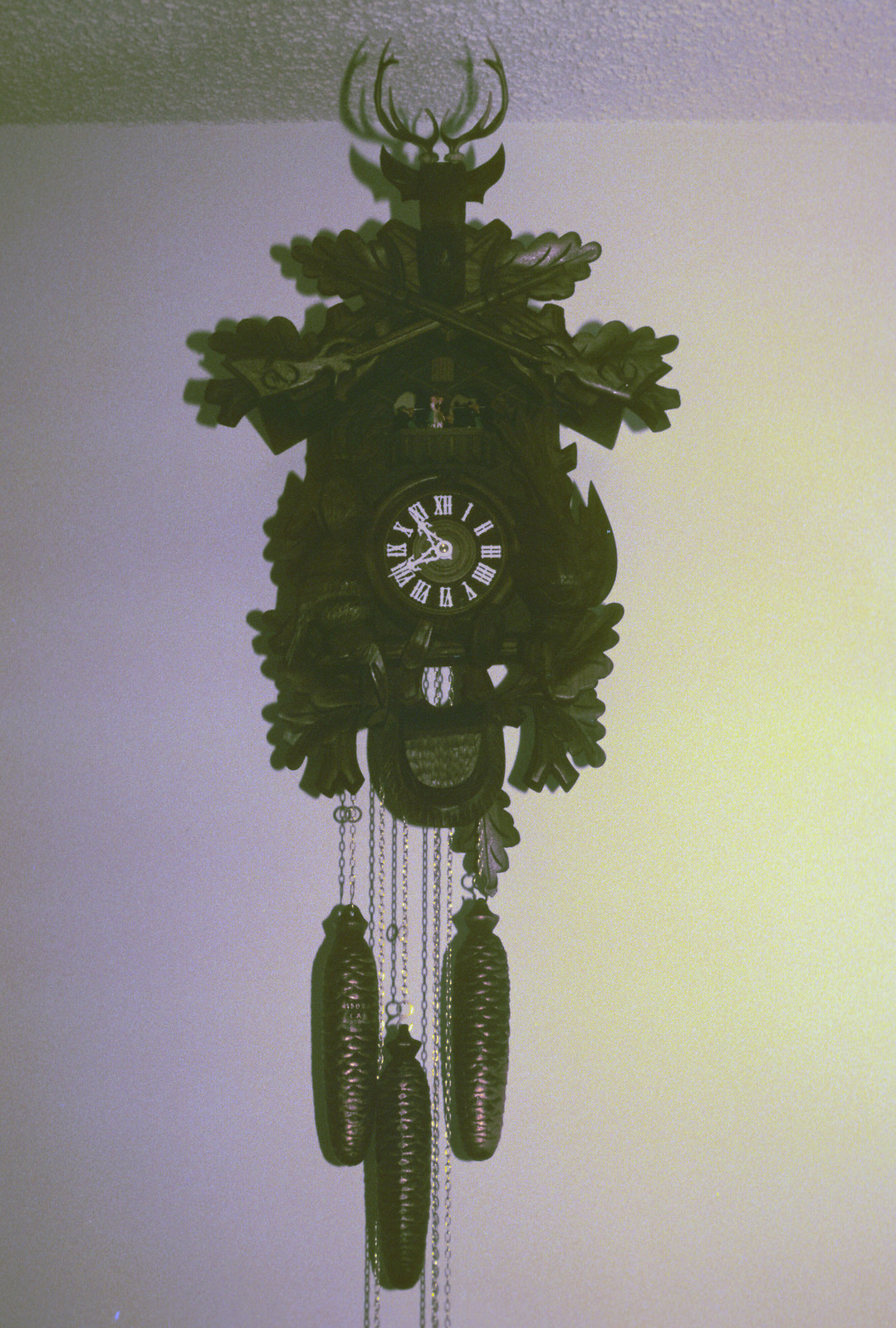The image depicts an intricately designed wall-mounted clock within a low-lit room that has a white textured ceiling and walls. This elaborate clock, reminiscent of Austrian or European craftsmanship, exudes a regal and old-timey aesthetic. The circular clock face is black with distinctly white Roman numerals from I to XII and matching white clock hands. The exterior of the clock is ornately decorated, resembling dragon scales and foliage, with features that evoke both plant-like leaves and elements of a dragon or animal wrapped around it.

At the very top of the clock, there are antler-like structures, suggesting a stag or nature-inspired motif, and intricate wooden carvings that resemble leaves with detailed etchings. Below these leaves, an opening hinting at a cuckoo clock mechanism is visible. Further down, three large, rectangular, pendulum-like structures or acorns hang from chains, likely designed to move or chime on the hour. The surroundings include a rough roof with scratch marks, adding to the image’s vintage atmosphere. The entire clock ensemble is black, enhancing its grand and dramatic presence in the room.